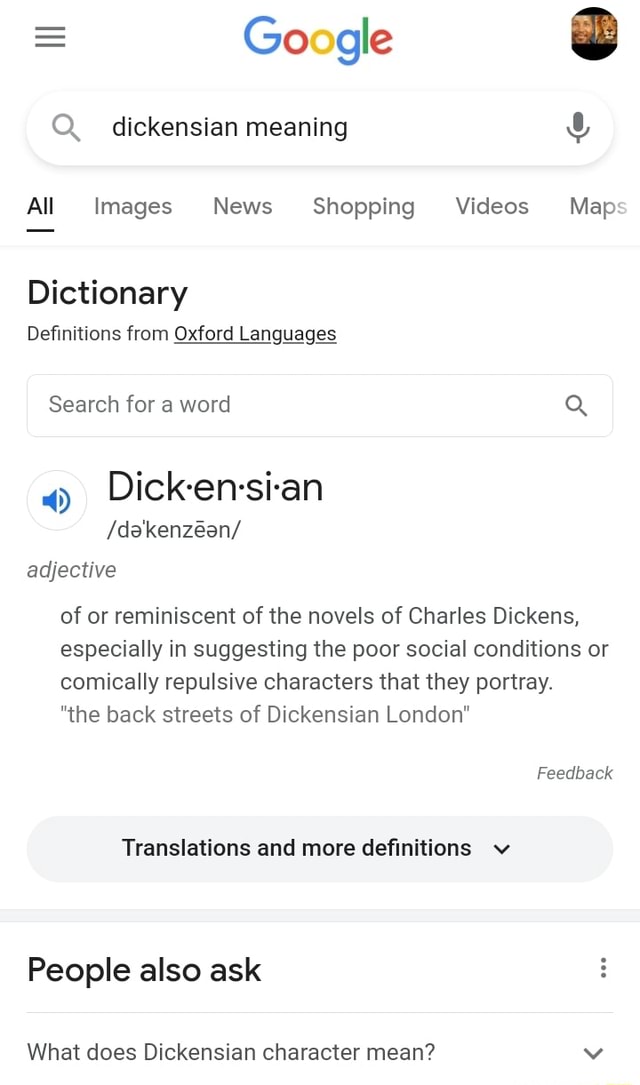**Caption:**

A detailed screenshot of a Google search page captured on a digital device, such as a desktop, laptop, tablet, or smartphone. 

**Description:**
On the right-hand side of the page, there is a user profile icon showing an African American man smiling beside a lion with a distinctive mane. The lion’s mane is a vivid mix of brown, red, orange, and brown hues, accentuated with black bands at the top and bottom, resulting in a cut-off, circular appearance.

At the top-left corner, there is a three-line menu icon in dark gray or black, indicative of the settings button. Centrally placed is the Google logo, comprising an uppercase blue "G," followed by a red "O," a yellow "O," a lowercase blue "g," a lowercase green "l," and a lowercase red "e." 

The search bar, which is oval-shaped with a gray magnifying glass icon on the left and a black microphone icon on the right, contains the text "Dickensian." Below the search bar, various search categories are listed: "All" (selected and highlighted in black with an underlining black line), "Images," "News," "Shopping," "Videos," and "Maps" (partially cut off), all in dark gray.

Beneath this, the word "dictionary" appears in bold black text. Following this are the words "definitions from," leading to "Oxford Languages" in smaller bold black text with an underline. A secondary search bar below this is rectangular, bordered in light gray, and prompts users with "search for a word" in dark gray text. To the right of this, a dark gray magnifying glass icon is displayed next to a white circle with a dark blue audio symbol.

The term "Dickensian" is broken down phonetically beside the search bar as "D-I-C-K dot E-N dot S-I dot A-N," with pronunciation guidance also provided in phonetic symbols: /ˌdɪkˈɛnziən/. Highlighted in italicized gray is the word “adjective.”

The definition provided states: "Of or reminiscent of the novels of Charles Dickens, especially in suggesting the poor social conditions or comically repulsive characters that they portray." An example within quotations follows: "The backstreets of Dickensian London."

To the bottom right, the word "feedback" appears in italicized gray. Directly below, there is a mid-gray, oval-shaped button with black text and a drop-down arrow reading "translations and more definitions."

Outside the main search results, the interface features a small, dark gray bezel and is divided by a light gray line into two white rectangles. The first rectangle offers bold black text, "People also ask," with a vertical trio of ellipses in gray for additional settings on the right. The second section poses the question, "What does Dickensian character mean?" indicated with a drop-down arrow.